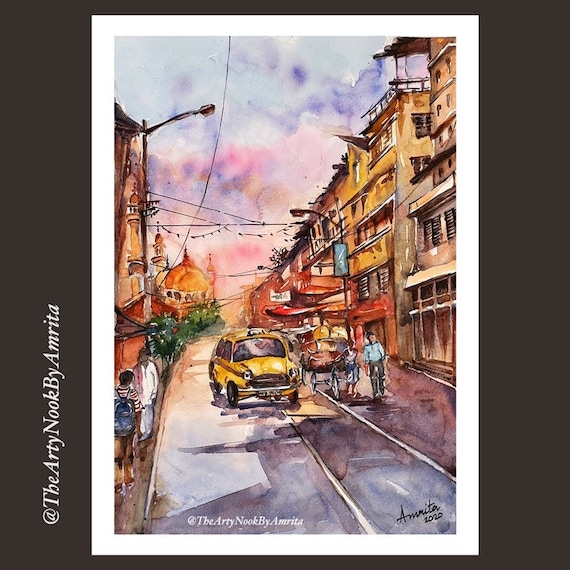This detailed painting titled "The Artie Nook by Amrita" features a vibrant, colorful cityscape framed by a dark gray background and white inner border. The painting, a square watercolor, depicts a bustling urban street lined with mid-sized apartment buildings that transition in color from light brown to yellow and then to orange. The street stretches into the distance, converging in the middle of the scene. A yellow taxi, shown head-on, drives down the center of the road, with cyclists riding alongside it. On the left side, pedestrians walk on the sidewalk next to lush green shrubbery and an enigmatic large orange object resembling a giant peach. On the right side of the street is a horse-drawn buggy. The buildings on the right appear somewhat disordered, in varied shades of gold, red, brown, and tan. The street itself is rendered in deep hues of black, blue, and purple. Above, the sky suggests a sunset with a mesmerizing blend of colors—light and dark blue clouds interspersed with shades of purple, pink, light orange, and gold. To either side of the street, various people add to the lively atmosphere of the painting.